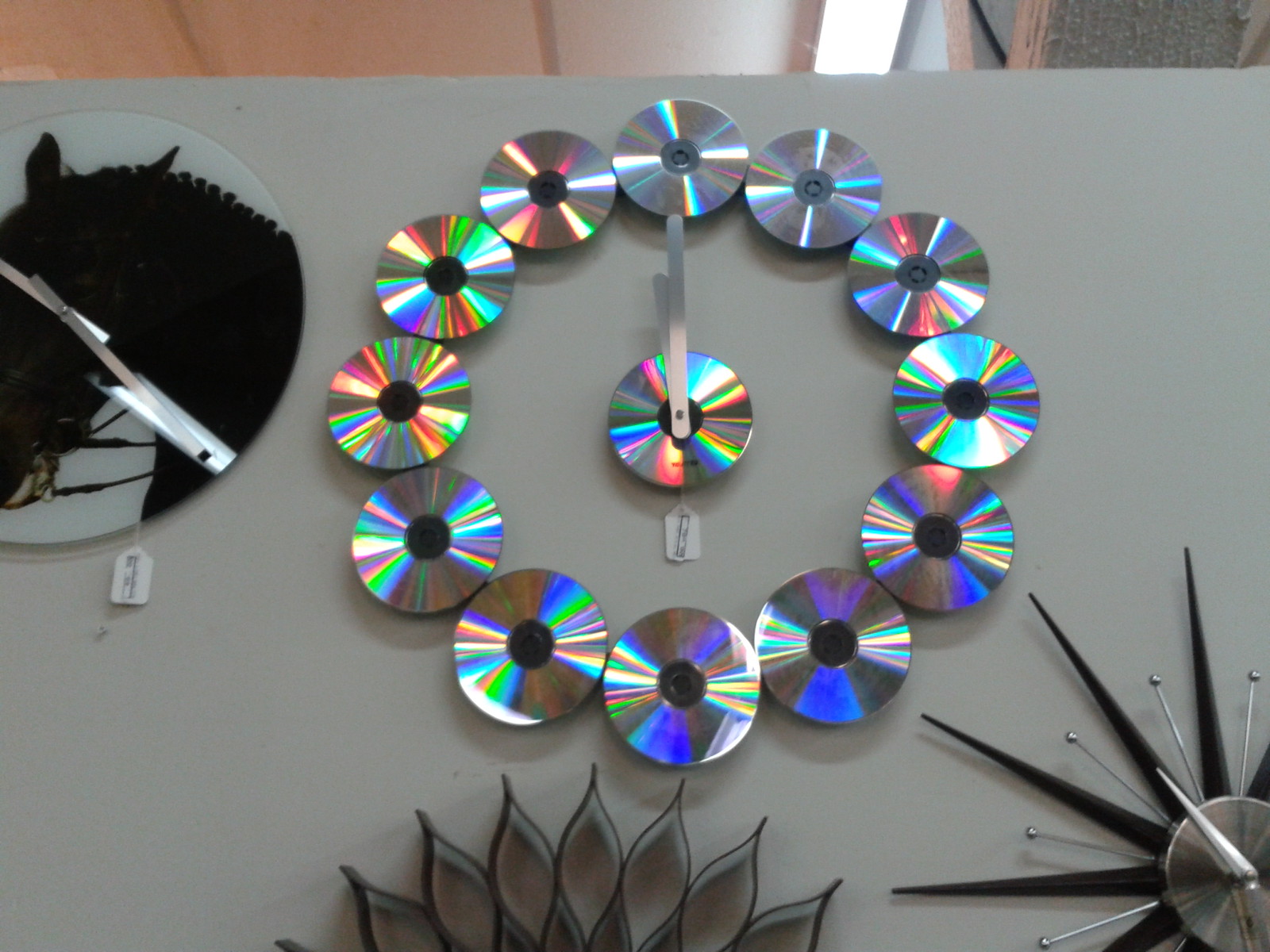The image appears to capture a display of several unique, artistically-crafted wall clocks within a shop setting. The background is a light-colored or white display wall. On the far left, there is a clock featuring a circular, shiny plastic or perspex disc with a black silhouette of a horse's head. Below this clock, there seems to be a price tag, indicating it's for sale. Dominating the center is an eye-catching clock made out of 12 holographic CDs arranged in a circle to represent the hours, with a central CD and silver metal hour and minute hands displaying a time just shy of 12 o'clock. To the bottom right, another clock is designed with black metal spikes extending outward like a star, interspersed with small rods ending in tiny silver balls, and a chrome silver face. Another clock below this has an outer frame shaped like flower petals, made of metal, further emphasizing the creative designs available for purchase in the shop.